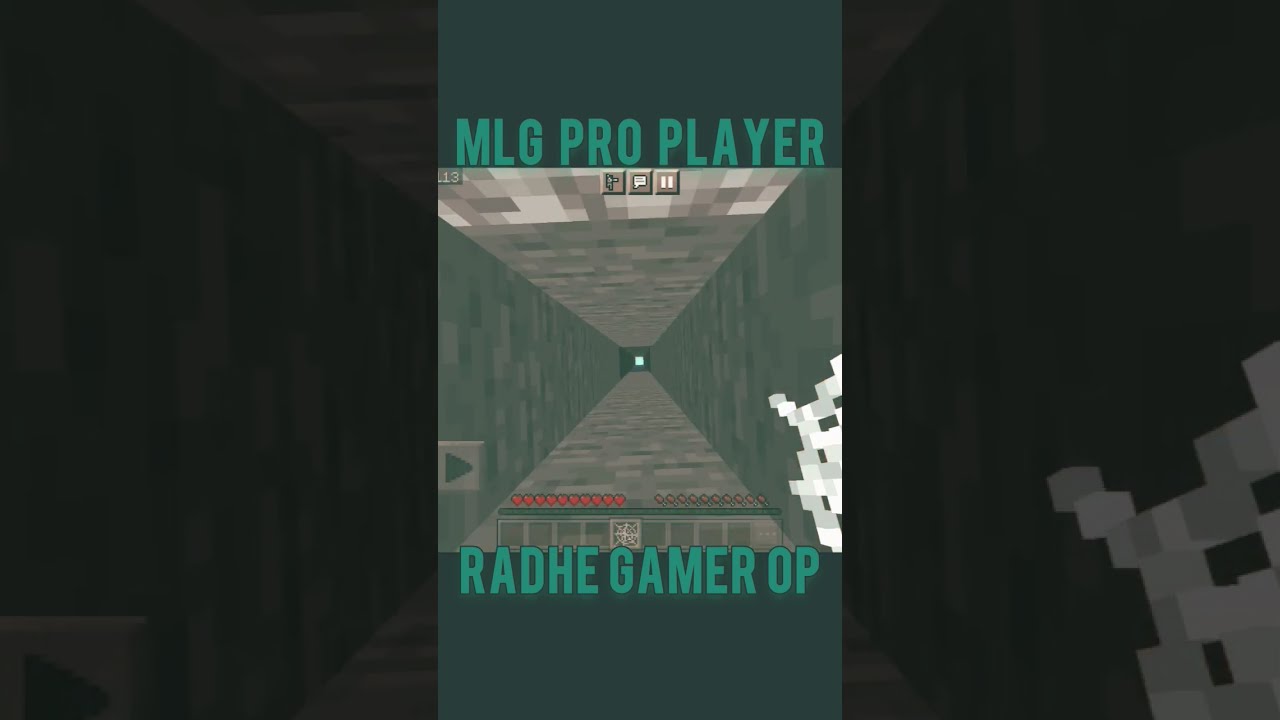The image is a detailed screenshot from a pixelated video game, resembling a tunnel or shaft with blocky, colored squares in gray, black, and green, reminiscent of retro games or Minecraft. The layout has three main sections: a central view down the "tunnel" surrounded by close-up panels on either side. At the top of the central section, the text "MLG Pro Player" is displayed in green capital letters, alongside three icons—a speech bubble, a pause button, and a figure of a golf player. Below the main tunnel image, more text reads "RADHEGAMEROP" in the same green, uppercase sans-serif font. The upper left corner features the number 13, while the lower left part shows a gray button with a black play arrow, beneath which there's a row of red dots, a row of gray dots, and a green line. The right close-up panel includes white squares indicating part of the tunnel’s wall, whereas the left panel has a close-up image of the play button. This screenshot likely captures a moment from a game, possibly during a streaming session by a player named RadHe.